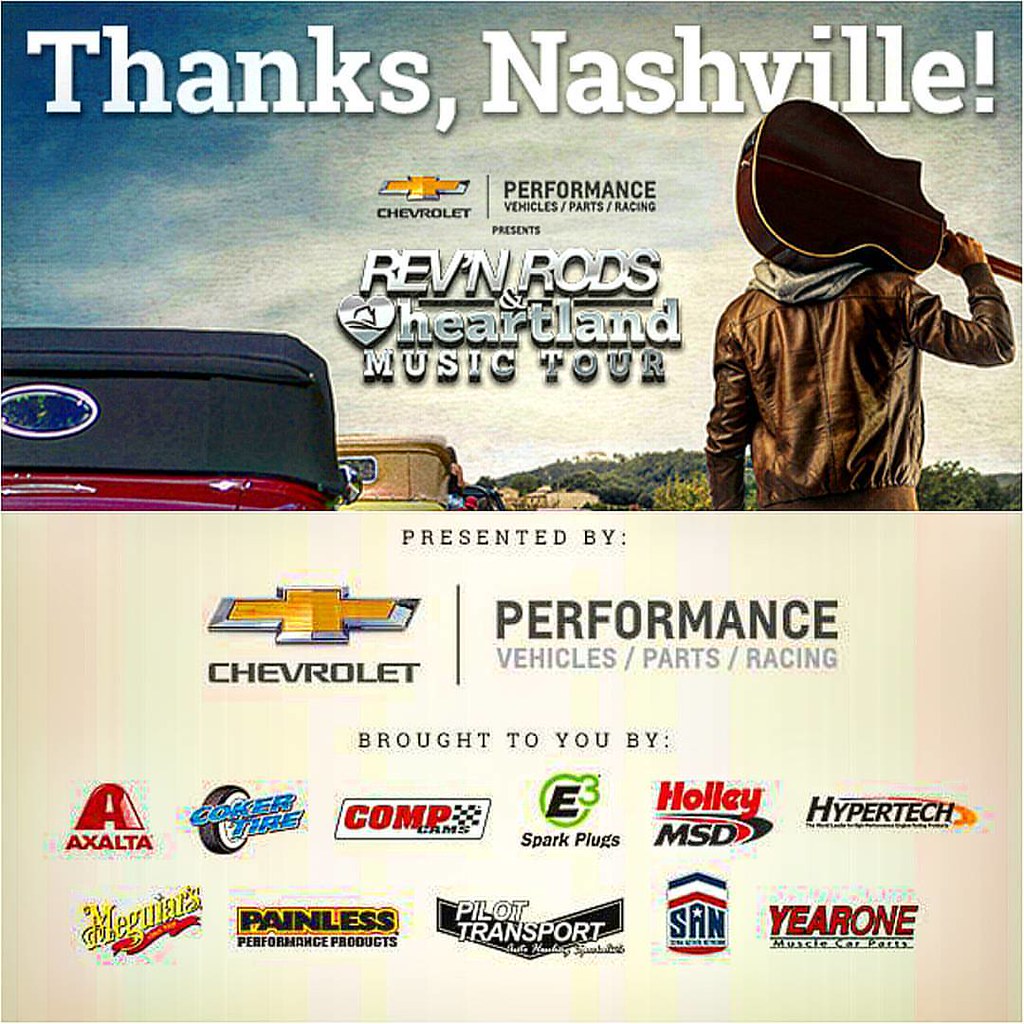The advertisement poster features a striking image in its top half, where a picturesque blue sky with scattered white clouds forms the backdrop. On the left side, there are several cars, possibly vintage models, adding a classic charm. To the right, a man with his back to the viewer carries a guitar slung over his right shoulder, creating a cool, laid-back vibe. Prominently overlaid on this background, the text reads, "Thanks, Nashville," in white, followed by "Chevrolet Performance Vehicles/Parts/Racing presents Revin' Rods and Heartland Music Tour," alongside a distinctive heart logo topped with a cowboy hat.

The bottom half of the poster transitions to a green background populated with various company logos. The text reads, "Presented by Chevrolet Performance Vehicles/Parts/Racing," followed by "Brought to you by," indicating the sponsors. The logos include well-known brands such as AXALTA, Coker Tire, Comp Cams, E3 Spark Plugs, Holley MSD, Hypertech, Mega Mars, Painless Performance Products, Pilot Transport, SAN, and Year One Muscle Car Parts, illustrating a broad base of industry support. The vibrant imagery, combined with detailed sponsor information, clearly positions this as a major promotional piece for the music tour.